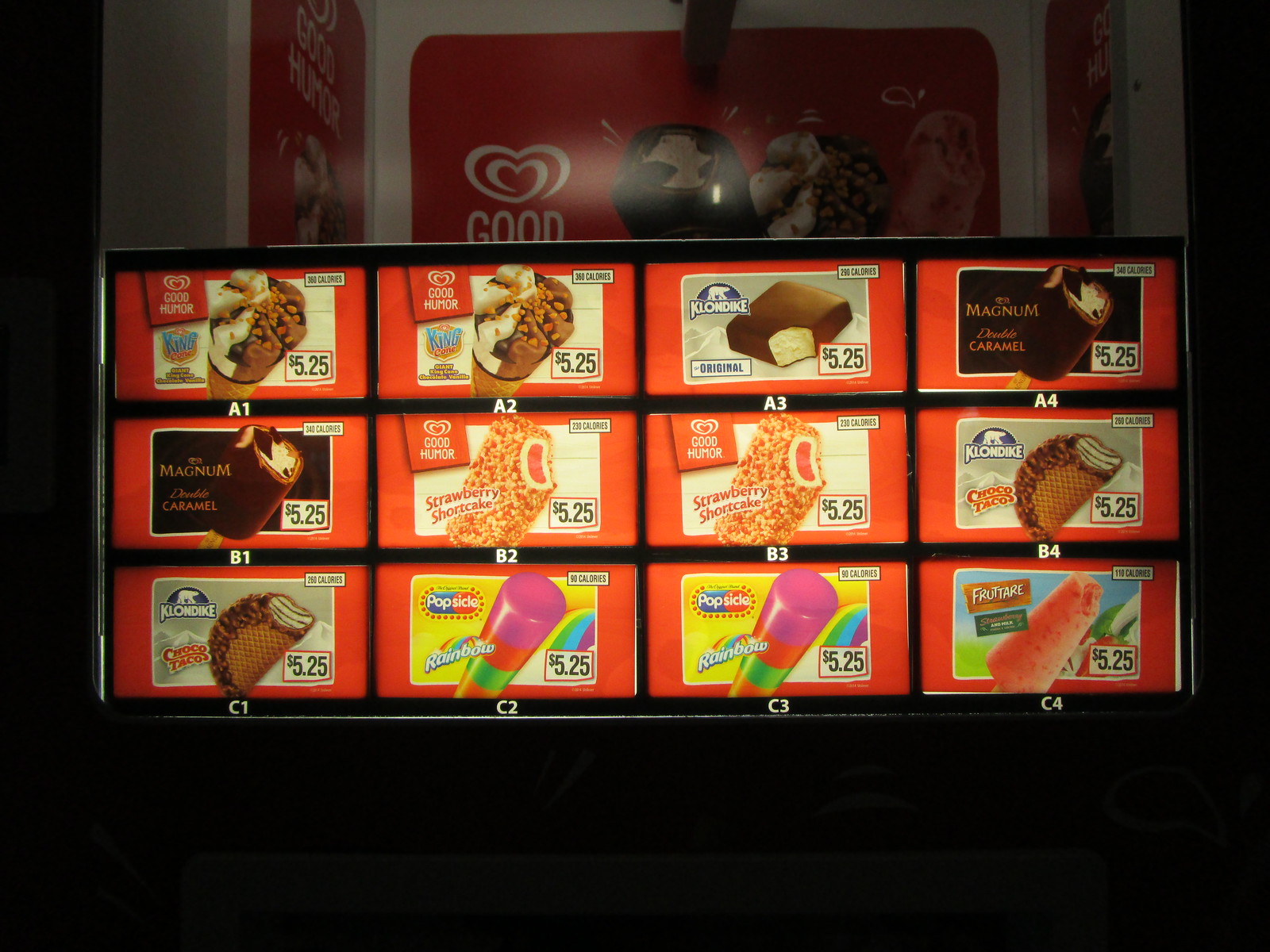The image captures a detailed display of an ice cream menu likely from an ice cream truck, set against a dark restaurant background. The centerpiece of the menu is a well-lit, backlit display featuring 12 ice cream novelties arranged in three rows with four items each, each item encased in a vibrant red border. At the top, the menu displays the Good Humor brand logo on a metal box-like structure, emphasizing the brand association.

The first row (A1 to A4) introduces the King Drumstick, another King Drumstick, a Klondike Bar, and a Magnum Double Caramel bar. All items are priced at $5.25 and include calorie counts, with the King Drumstick and Magnum Double Caramel both featuring 300 calories, and the Klondike Bar at 290 calories.

In the second row (B1 to B4), you find the Magnum Double Caramel again, followed by two Good Humor Strawberry Shortcake bars and a Klondike Choco Taco. Each item remains priced at $5.25, with the Strawberry Shortcake featuring 200+ calories and the Choco Taco described as a waffle cone shaped like a taco, filled with vanilla ice cream and chocolate, and topped with nuts.

The third row (C1 to C4) mirrors the second row initially with another Choco Taco, then transitions to colorful popsicles and another fruit-themed popsicle. The rainbow popsicle (C2 and C3) boasts vibrant stripes of pink, red, green, and orange, at 90 calories each, while the fruit-themed popsicle (C4) is an orangish-red frozen treat, concluding the menu with a consistent price of $5.25.

Overall, this organized and colorful menu provides a clear and tempting overview of various frozen dessert options, each distinctly marked with letters and numbers, and framed to catch the eye against the dimmed surroundings.